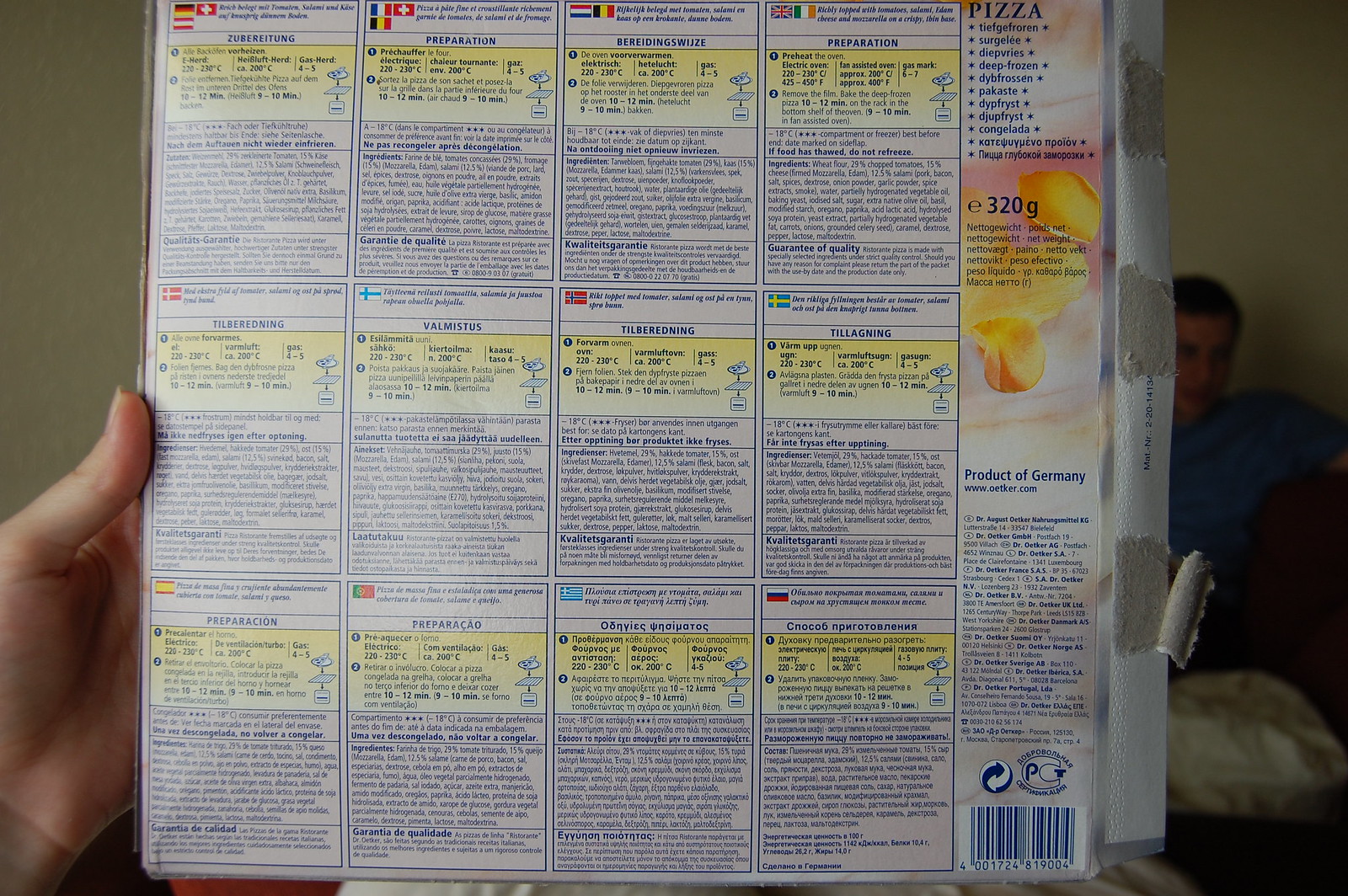This photograph showcases a left hand holding a sheet of paper filled with an abundance of text written in a foreign language. The paper is divided into approximately 12 squares, each featuring text predominantly in blue on a white background, with some sections displaying blue text on a yellow background. The top row of squares includes various flags of different countries. On the right side of the paper, the word "Pizza" is prominently written in blue letters at the top, followed by additional foreign language text. Below this, the phrase "Product of Germany" is printed. At the bottom right corner, there is a barcode.